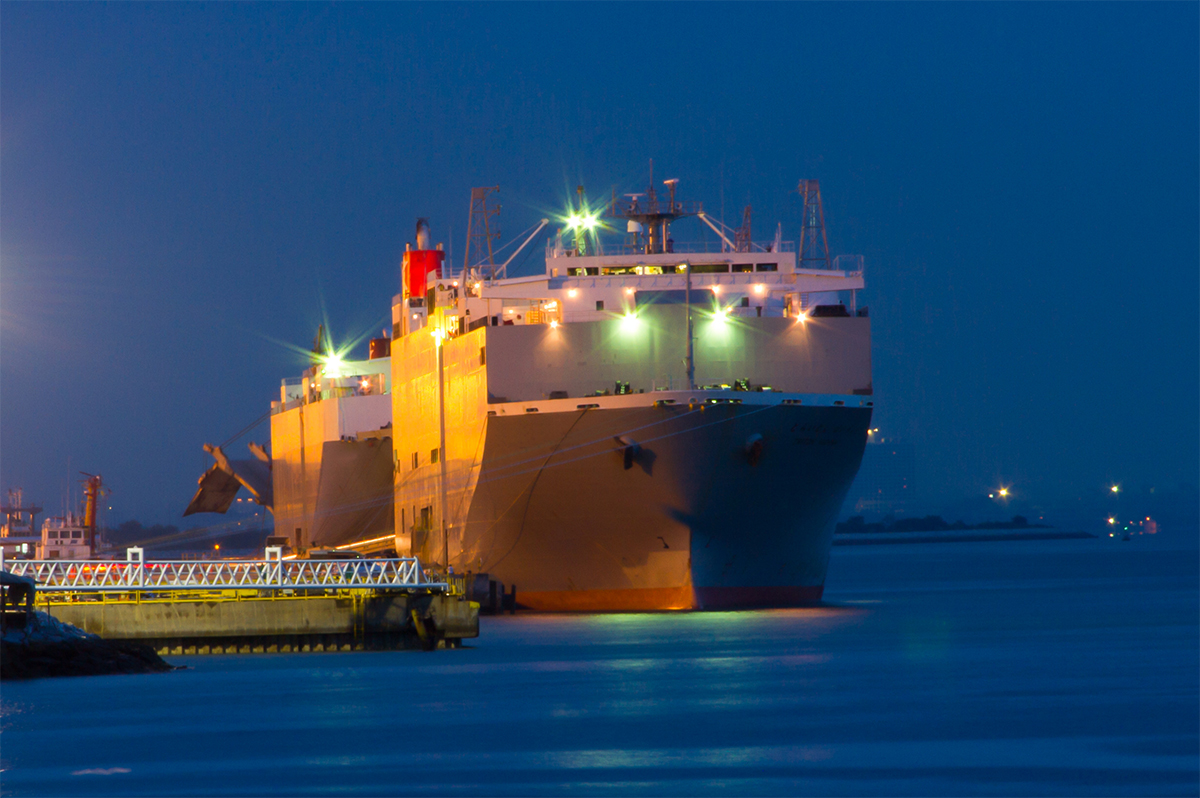The image, taken at night, depicts a large, heavy-looking ship possibly functioning as a cargo vessel. The ship is positioned primarily on the left side of the frame, floating on calm, blue water that reflects the bright lights from the vessel. The ship appears to be half yellow and half dark blue, possibly due to the lighting rather than its actual colors. The upper part of the ship is adorned with several green lights clustered together and more spaced out orange lights. There are distinctive features like a red square on the top side and what seems to be pieces of scaffolding extending from the left. Additionally, toward the front, there's a smaller yellow boat or dock with a white guardrail painted yellow. The backdrop includes a mountainous landscape with silhouetted trees and a faint light source, possibly from the moon or distant structures, along with towers further in the background. Towers and assorted lights across the scene contribute to the reflections in the water, adding to the image's intricate details.